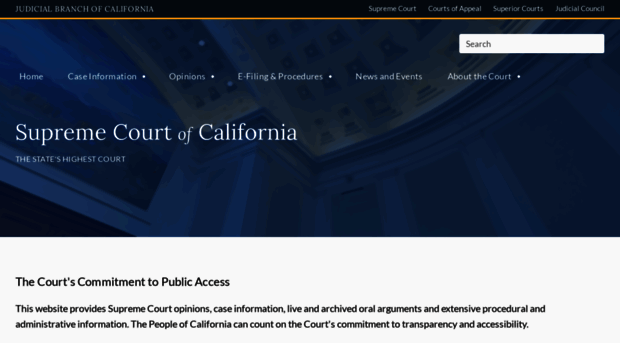A detailed screenshot of the Judicial Branch of California’s website features a black header that reads "Supreme Court, Courts of Appeal, Superior Courts, Judicial Council.” Below this header lies a gold bar. On the right-hand side of the page, there's a white search bar. The website navigation includes links labeled "Home," "Case Information," "Opinions," "E-Filing and Procedures," "News and Events," and "About the Court." The center of the page states "Supreme Court of California" in white letters, designating it as the state's highest court. The main focal point is a high-quality image taken from a low angle, showcasing the ornate courtroom. Light-colored wood paneling lines the walls, and the ceiling, adorned with detailed artwork, is gently illuminated. The image conveys a nighttime ambiance, with pillars adding to the grandeur of the scene.